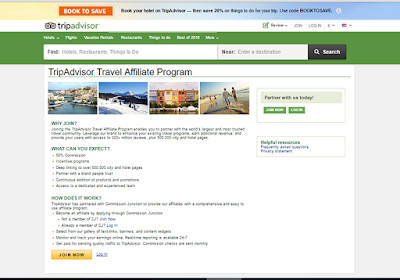Here is a more detailed and cleaned-up version of the caption you provided:

---

The screenshot showcases a low-resolution image of a website, likely TripAdvisor. At the top, there is a horizontally aligned, multicolored pastel bar transitioning from pastel yellow on the left to pastel purple on the right. Resting within this bar on the left is an orange rectangle with the text "BOOK TO SAVE" in white font. Adjacent to this, in black font, is a promotional message: "Book your hotel on TripAdvisor – and save 20% on things to do on your trip! Use code BOOK TO SAVE."

Additionally, there is a small white circle containing a black exclamation point.

Below this pastel bar, a white rectangular section features the TripAdvisor logo, consisting of an icon resembling binoculars. The text "Trip" appears in black font next to "Advisor" in red font.

On the same pastel bar, to the right, are clickable options for changing the website language and user login.

Underneath this section is a prominent red rectangle containing a white search field for site-wide queries. Next to this search field, there is placeholder text prompting users to "Enter a destination" near the term "NEAR."

---

This detailed description captures the visual elements and layout of the website screenshot, making it easy to visualize and understand.